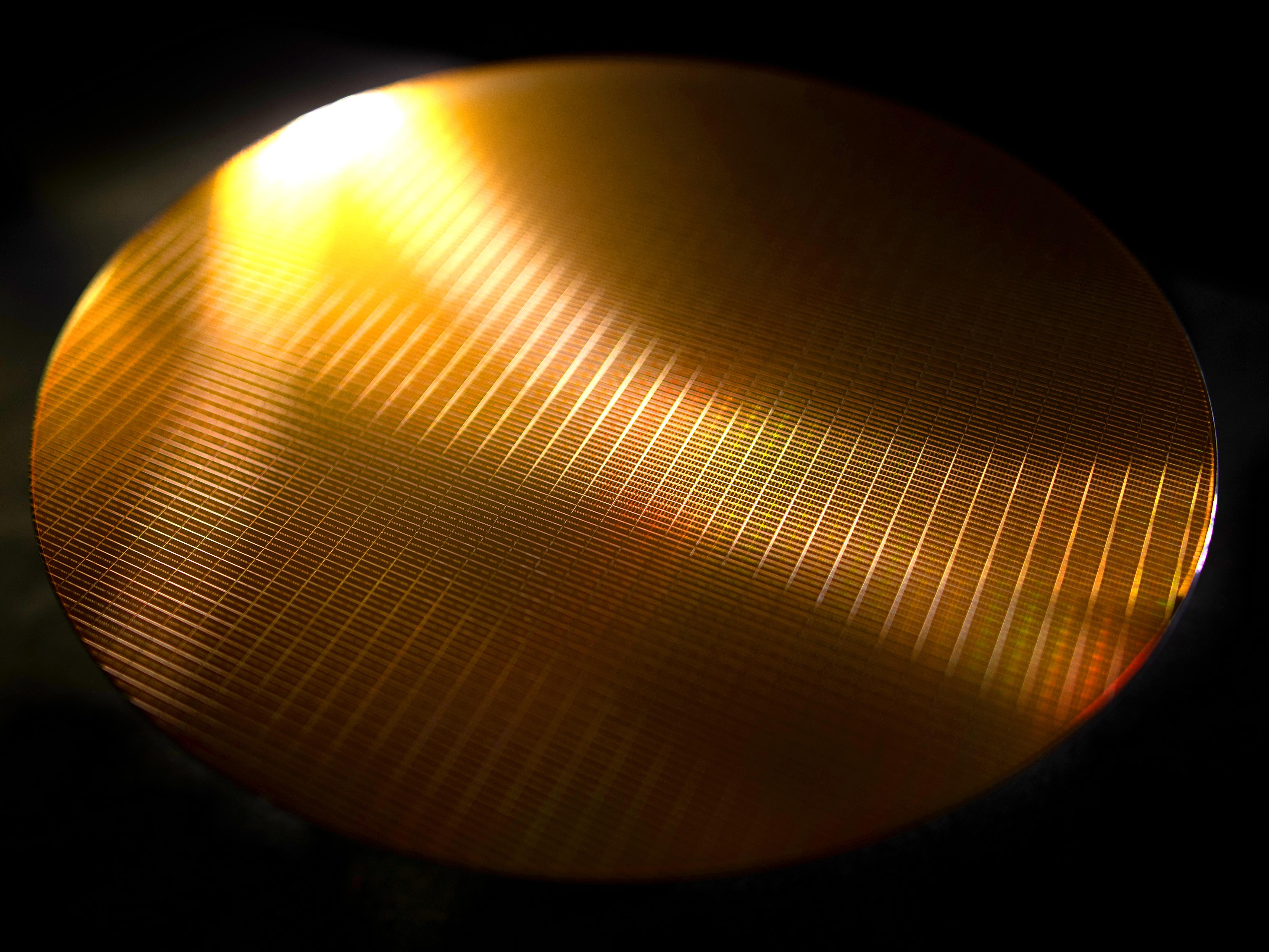The image features a sophisticated, flat, circular disc with a brassy gold hue, situated against a completely black background. The disc appears to be metallic and has a detailed grid pattern composed of small squares or rectangles. Light from the top left corner casts a band of illumination across the object, creating a multi-colored reflection that gives the surface a complex, shimmering appearance. Despite its intricate design, the purpose of the disc remains ambiguous, resembling a computer chip, a filter, or even a decorative piece. The overall presentation is minimalistic, with no additional text or markings, emphasizing the disc's refined and enigmatic nature.